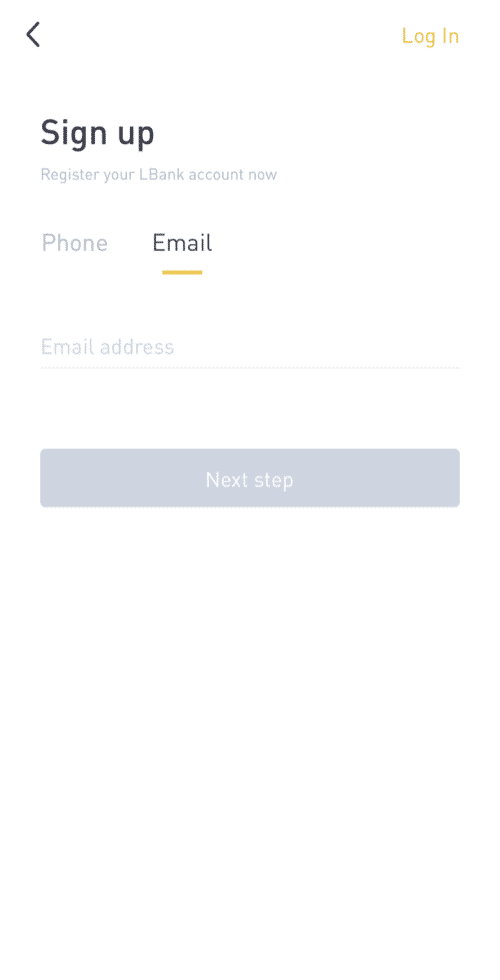A very minimalistic registration page for an LBank account is captured in this image. The interface features a predominantly white, vertically oriented rectangular layout. In the top left corner, there is a small left-pointing arrow. To the right at the top, the word "Login" appears in yellow, while directly below on the left side, "Sign Up" is written in bold black. Further down, the text "Register your LBank account now" is displayed in gray. 

Beneath this prompt, there are two options: "Phone" in gray and "Email" in black, with a yellow underline indicating the active selection. Below this is a light gray line, accompanied by the placeholder text "Email Address" in gray above it. The lower section of the page includes a large, horizontally extended white rectangle outlined with a gray line, featuring the text "Next Step" centered within it. 

The design utilizes a color scheme of black, white, gray, and yellow. The spacious layout devotes a substantial portion of the screen to blank white space, creating a sparse and uncluttered look. This screen could be displayed on various devices, such as a phone, tablet, or computer, but the exact platform is unclear due to insufficient context.